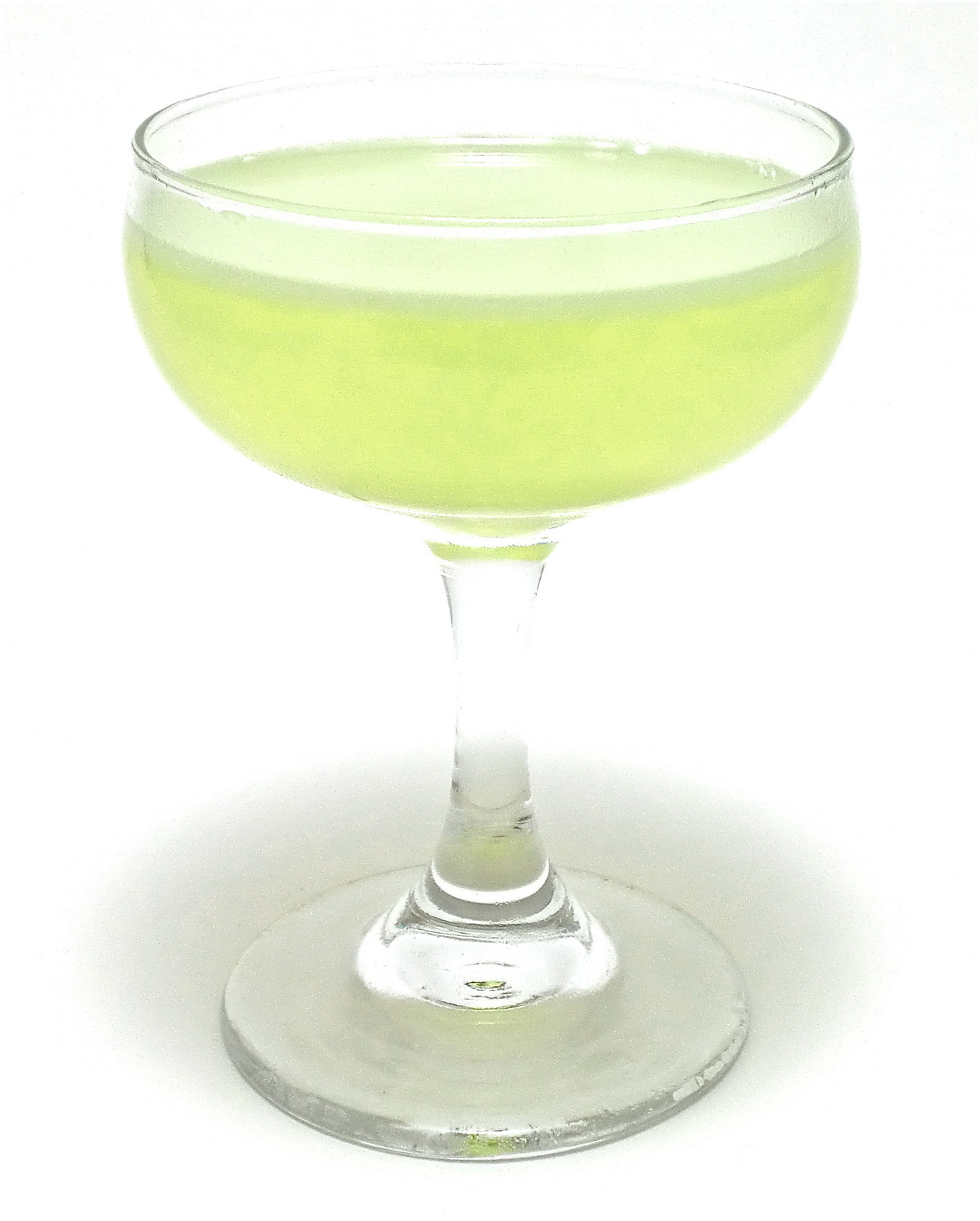This image features a clear, stemmed glass reminiscent of a margarita or champagne glass, characterized by its rounded bottom and broader, shallower bowl at the top—the glass narrows at the stem and flares out again towards the top. It is filled three-quarters full with a yellowish-green liquid, possibly a cocktail like a margarita or white wine, notable for its plain appearance without any embellishments like salt on the rim. The glass casts a shadow suggesting it is placed on a flat surface; however, the absence of a visible table and the uniform white background give an ambiguous context—hinting that it could be a photograph, digital artwork, or a painting. The shadow around the base of the glass adds a realistic depth to the scene, reinforcing the idea of a physical presence within an abstract or minimalistic setting.